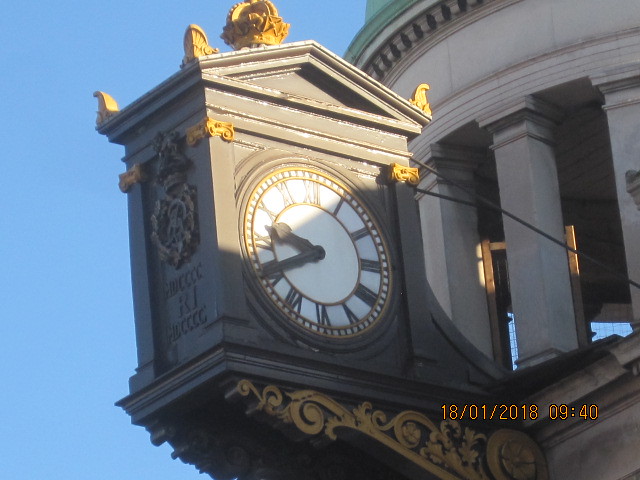The photograph, dated January 18, 2018, at 9:40, captures a stunning scene dominated by a clock tower under a clear, vibrant blue sky. The structure, likely made of white concrete or marble, features tall, pristine white slabs or columns. The focal point of the image is the intricately designed clock. The clock, set within a brown frame adorned with delicate golden designs, has a cream-colored face. Dark brownish-black Roman numerals mark the hours, with matching dark hands indicating the time. The photo beautifully juxtaposes the classical elegance of the clock tower with the modern clarity of the date and time stamp in the bottom right corner.